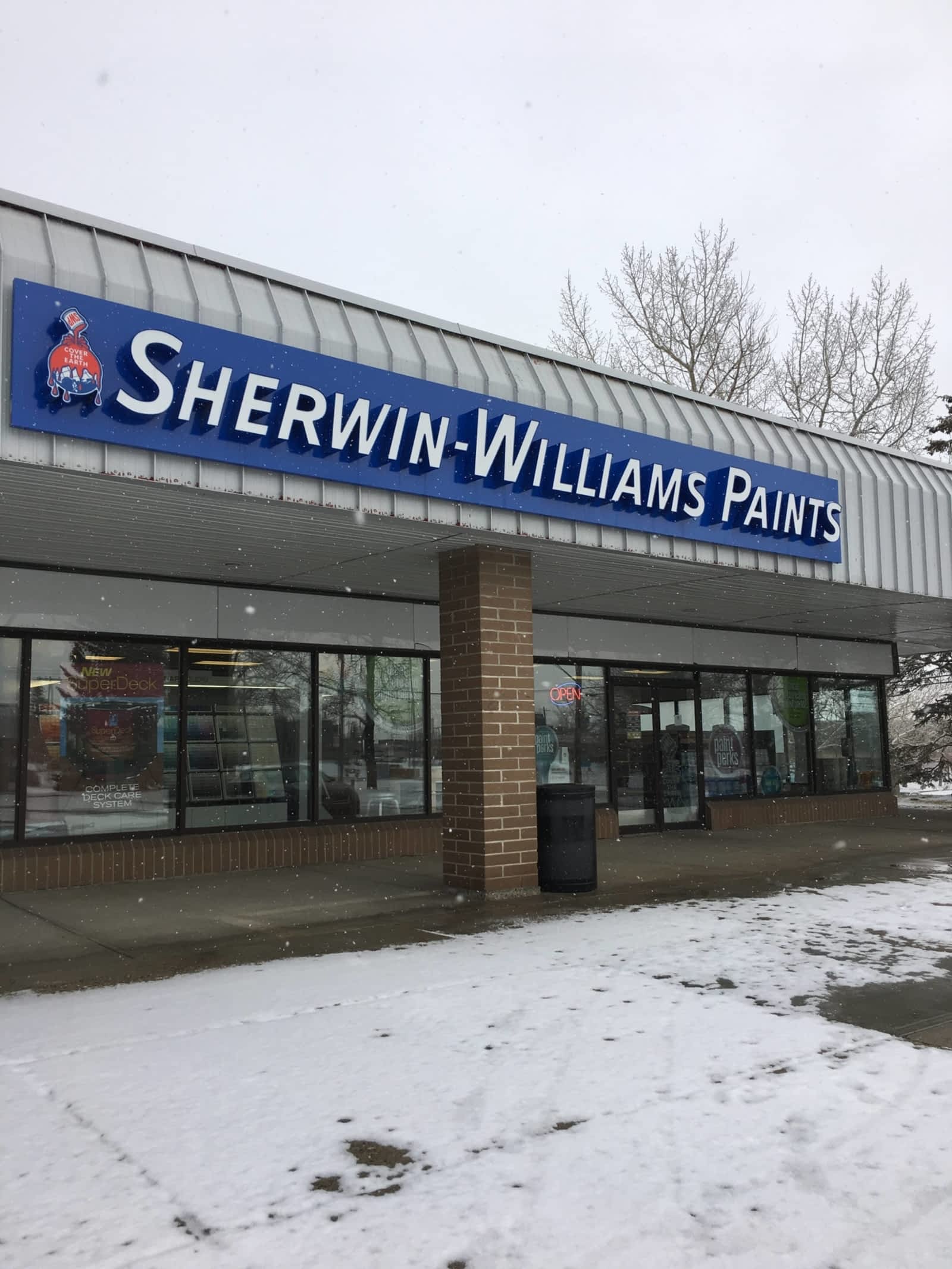This image showcases a Sherwin-Williams Paints store, prominently featuring a blue sign with white lettering. The primarily brick building is complemented by off-white ceiling panels, creating a stark yet pleasing contrast. The entrance to the store is made up entirely of glass windows, providing a clear view inside. Adjacent to a brick pillar, a trash bin is visible, adding to the everyday scene.

Snow blankets the ground and dusts the air, contributing to a serene, wintry atmosphere, further emphasized by the absence of cars and people. An illuminated 'Open' sign in the window signals that the store is ready for business, despite the weather. In the background, leafless trees and branches stand in silent witness to the season. The photograph appears to have been taken from outside, capturing not only the building's façade but also the peaceful winter setting.